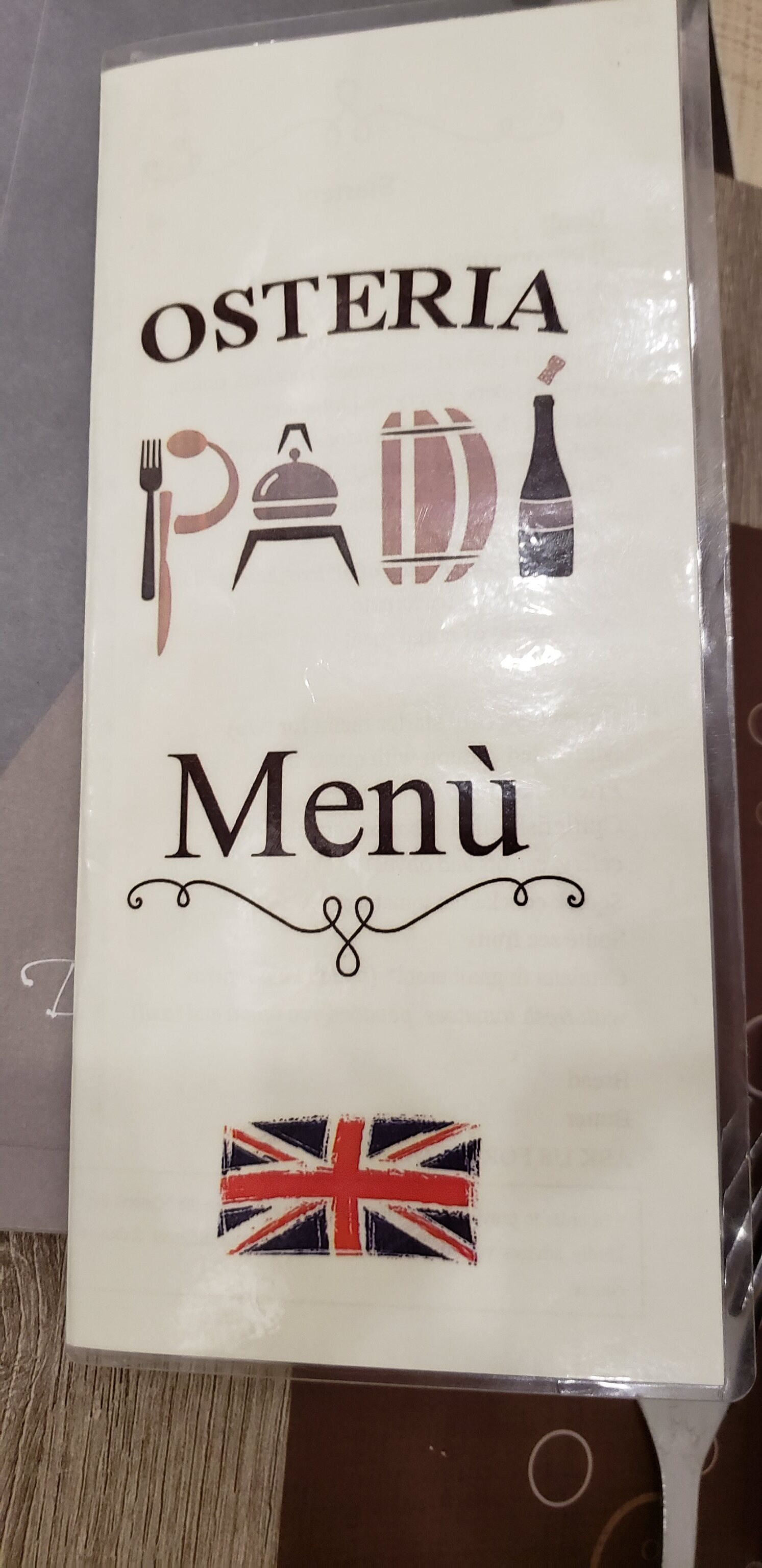The image features a tall, vertically rectangular menu situated on a light gray wooden table accented with a light gray and almost white light blue tablecloth. The menu, which is off-white and encased in a clear plastic lamination, prominently displays the text "Osteria Menu" in black at the top center. Positioned beneath the title from left to right are a series of illustrative icons: a fork, an unusual utensil resembling an egg topper with a curved handle and egg-shaped tip, and a rounded pot on a burner with a small handle at the top. Further to the right, the icons continue with a partial image of a wooden barrel and a wine bottle. Below the word "Menu" is a decorative swirl, and centrally placed at the bottom of the menu is the British flag.